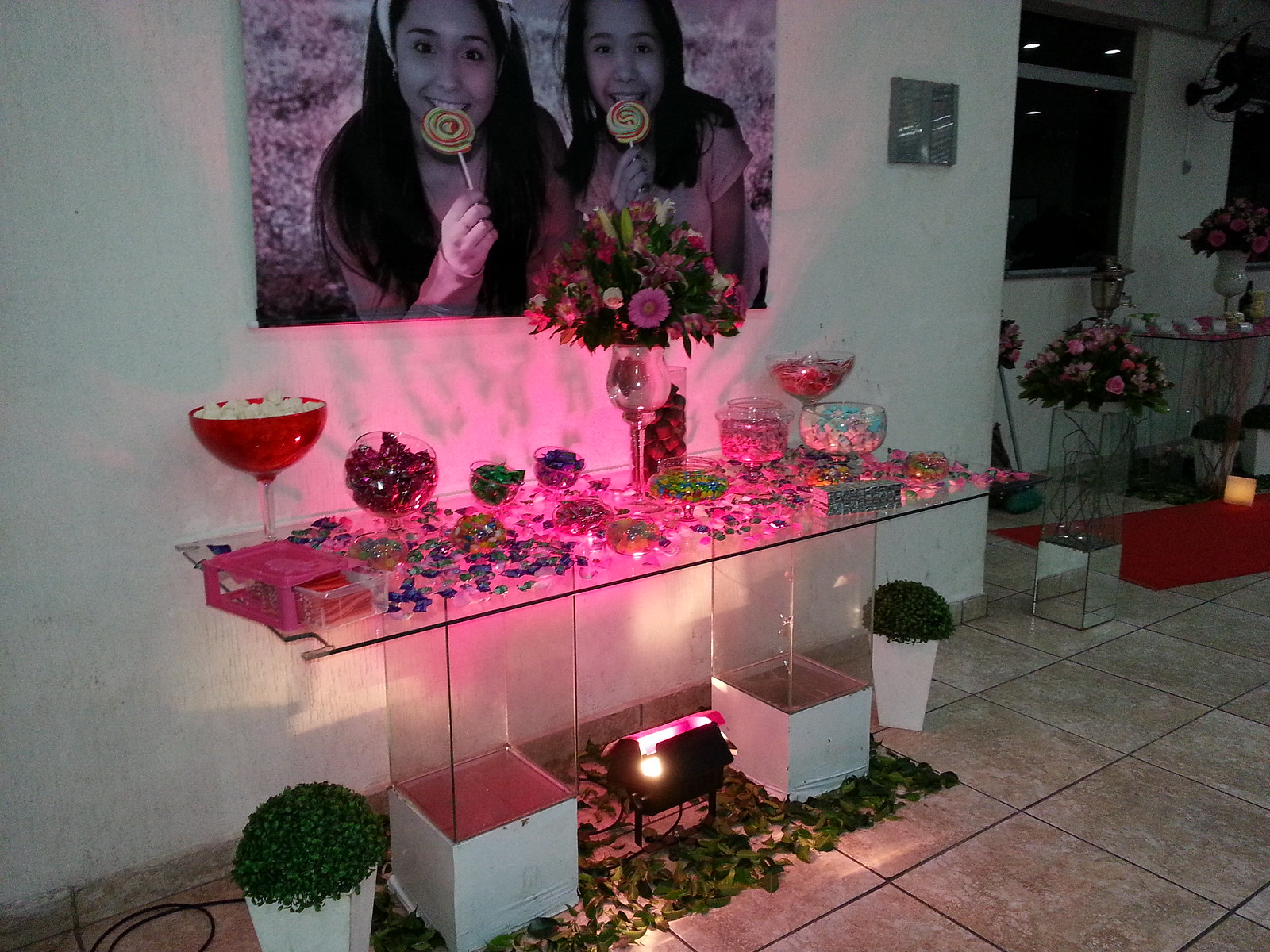The photograph captures a lively and vibrant party scene set against a whitewashed wall. Central to the image is a sleek glass table adorned with a variety of snacks and colorful candy. Numerous glass jars and bowls of varying sizes are filled with candy wrapped in vibrant hues of red, blue, purple, and pink, spilling over onto the table itself. Among the confections, a prominent bowl brims with flowers. Nestled in the middle of the table is a vase filled with an additional bouquet of flowers, bringing a touch of natural beauty to the spread.

On the wall behind the table hangs a striking monochrome photograph of two girls enjoying lollipops—the only elements in vivid color—one older and the other younger, the latter positioned to the right. Both girls are captured mid-lick, adding a playful and nostalgic touch to the scene. The floor is tiled and features additional green plants, along with another bouquet of flowers positioned on the right side of the image, contributing to the whimsical and festive atmosphere.